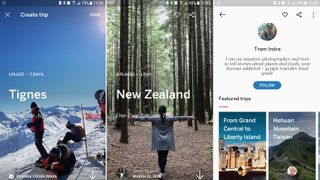The image consists of a vertical collage of three distinct screenshots from a person's phone, possibly depicting an app they were using. 

- **Left Image:** This screenshot captures a snowy mountain landscape under a clear blue sky. Two men are standing, clad in full winter gear - including heavy winter coats, black pants, and black hats. Skis are visible, indicating they are likely skiing. Above them, in white text, reads "TIGNES," suggesting the location is Tignes, a ski resort in France.
  
- **Middle Image:** The central screenshot portrays a serene forest path flanked by tall, dark brown or black trees, their tops adorned with lush green leaves. The ground is covered in brown leaves, signifying autumn. A woman, shown from behind, stands on the path with her arms extended horizontally, forming a cross-like shape. She has long black hair and is dressed in black pants and a gray shawl or jacket. Above her, the white text "New Zealand" denotes the location.
  
- **Right Image:** The final screenshot has a white background featuring a small avatar image of a person, possibly a woman of European descent. Beneath the avatar, in black, is the text "Team" and a name, likely "Tirum Limdra" though it's difficult to decipher. A blue box with the word "Follow" in white is positioned horizontally. Below this, there are two small images: one depicting the New York City skyline as seen from the water, with the text "from Grand Central to Liberty Island," and the other related to the "Hawoon Mountains."

This detailed collage captures diverse locations and activities, from snowy mountains and serene forests to urban landscapes and possibly social media interactions.